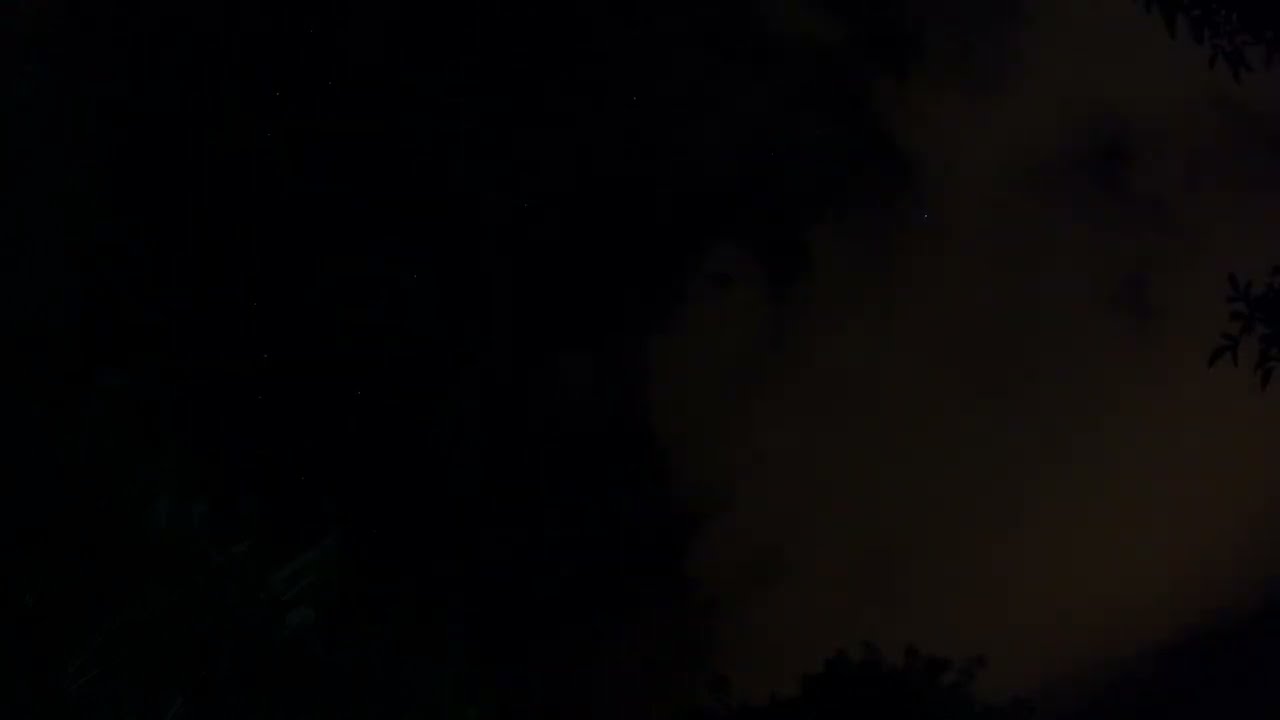The image is an extremely dark, rectangular expanse, predominantly solid black with some subtle variations. Within this largely monochromatic composition, there is a slightly lighter gray area off to the right-hand side, occupying approximately one-third of the image, which might suggest clouds in a night sky or a frosty window, though it remains ambiguous. The remaining portion of the image is entirely black, with no discernible details. It is unclear whether this is a technical issue, a blank slide, or an intentional artistic choice.